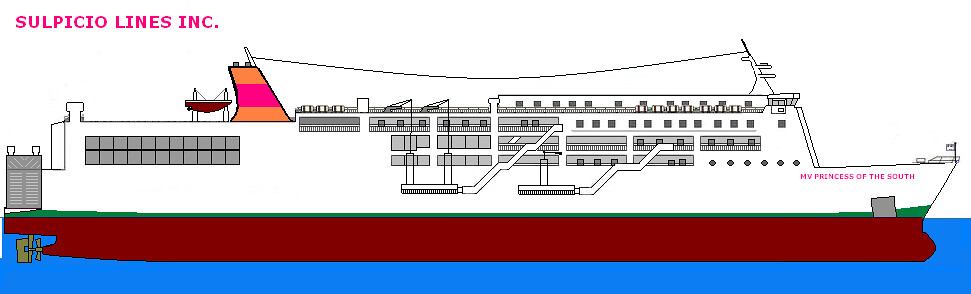This digital artwork showcases a side profile of a three-story cruise ship rendered to sit in a blue body of water. The vessel belongs to "Sulpicio Lines, Inc." as indicated in a pink font on the top left corner of the image. The ship's name, "MV Princess of the South," is prominently displayed on the right side. The hull of the cruise ship is burgundy, while the upper structure is entirely white. A distinctive feature is the ship's orange tail fin adorned with a pink and orange stripe, situated toward the rear, which is also where lifeboats are located. The ship is equipped with an olive-colored propeller and a large engine block at the very back. Several staircases connect the lower decks to the top deck, near the captain's main quarters, emphasizing the cruise ship's three-story design. The black part of the ship below the waterline contrasts sharply with the vibrant colors above, capturing a simple yet detailed depiction of the vessel.